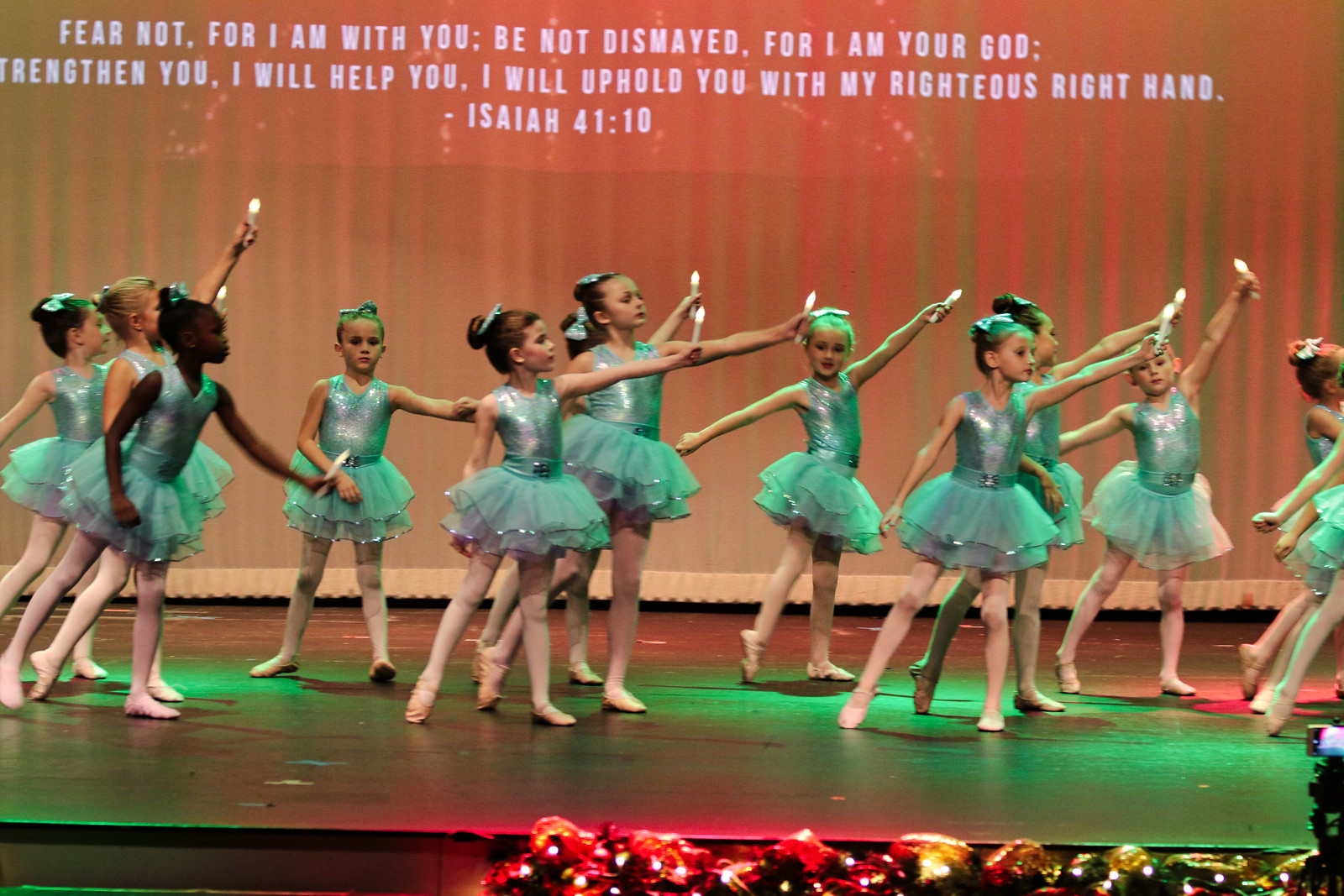In this captivating photograph, a group of young girls, likely in the early years of elementary school, stand or dance on a stage, performing as ballerinas. They are dressed in matching light blue, almost teal tutus with sleeveless, tight-fitting tops and sheer skirts, complemented by white tights and pink ballet slippers. Their hair is neatly tied up in buns adorned with matching teal ribbons. Each girl holds aloft a white candle with an LED bulb, casting a delicate light.

The stage is a flat, black surface bordered at the bottom by a festive garland of greenery interwoven with red and yellow Christmas lights, adding a whimsical touch to the scene. A greenish spotlight enhances the ethereal atmosphere. 

The backdrop is a white curtain onto which a powerful Bible verse from Isaiah 41:10 is projected in white, sans-serif text: "Fear not, for I am with you; be not dismayed, for I am your God. I will strengthen you, I will help you, I will uphold you with my righteous right hand." This inspiring message looms over the girls, adding a profound sense of grace and encouragement to the performance.